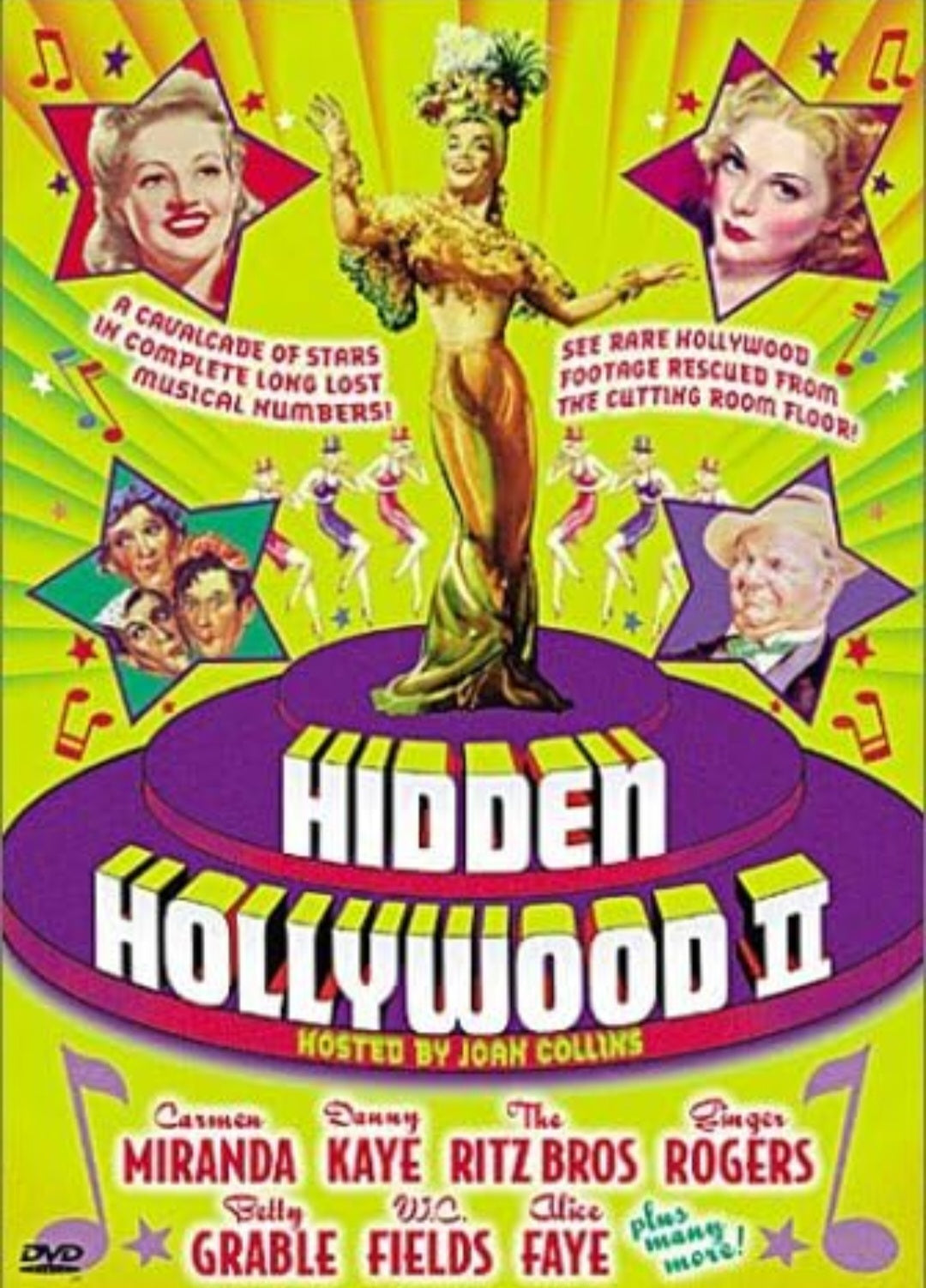The cover of the DVD for "Hidden Hollywood 2, hosted by Joan Collins," captures the essence of 1930s and 1940s Old Hollywood with its illustrated effect. The background features bright lines of yellow fading into green at the bottom. Central to the cover is Carmen Miranda, standing on a three-tiered purple platform. Prominently displayed in large white letters is the title, "Hidden Hollywood 2, hosted by Joan Collins," beneath which the names of classic Hollywood stars are listed in red: Carmen Miranda, Danny Kaye, The Ritz Brothers, Ginger Rogers, Betty Grable, W.C. Fields, and Alice Faye, with a note in teal promising "plus many more."

In the upper left-hand corner, a red star features Betty Grable, while on the upper right-hand side, another red star showcases Ginger Rogers. Below, in the left corner, a teal star contains the Ritz Brothers, and a purple star on the right displays W.C. Fields. The poster's elaborate design includes an array of musical notes and stars, bringing a lively, nostalgic feel to this homage to hidden Hollywood gems.